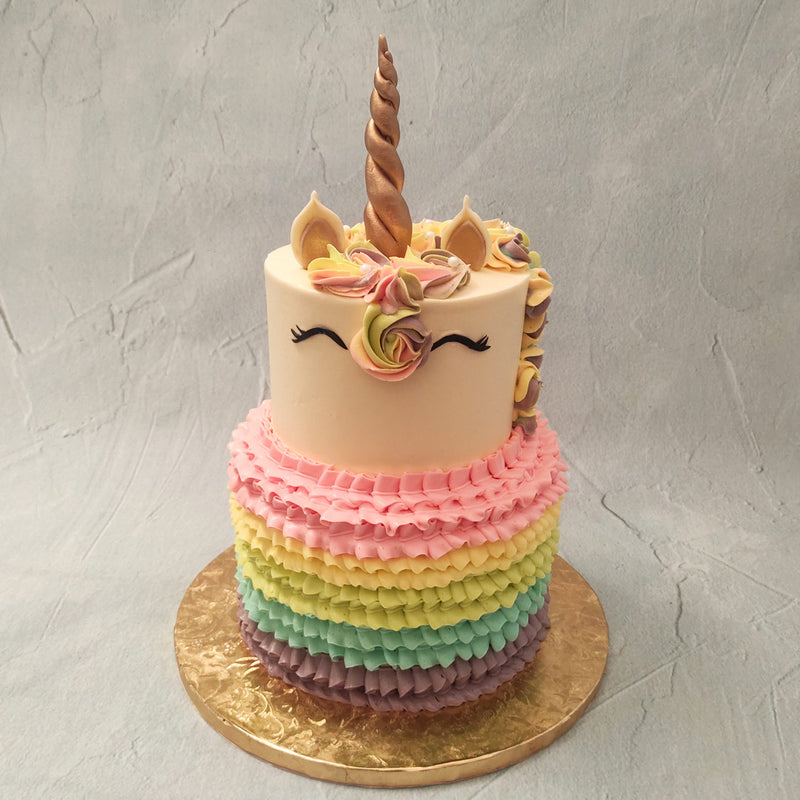This photograph showcases a beautifully intricate unicorn-themed birthday cake set against a gray and white plaster background. The cake is prominently placed in the center on a round, golden-painted wooden tray. The bottom half of the cake features layers of frilly icing in vibrant shades of pink, yellow, green, teal, and purple, creating a visually appealing and dress-like pattern. The upper portion of the cake is a smooth, white surface adorned with delicate black lines forming the unicorn's eyes. Topping the cake are a pair of ears and a golden horn, surrounded by a mane crafted from rose-patterned frosting that cascades to the side. The overall presentation suggests the cake is likely intended for a child's birthday celebration and has been meticulously styled, potentially for social media or promotional purposes.